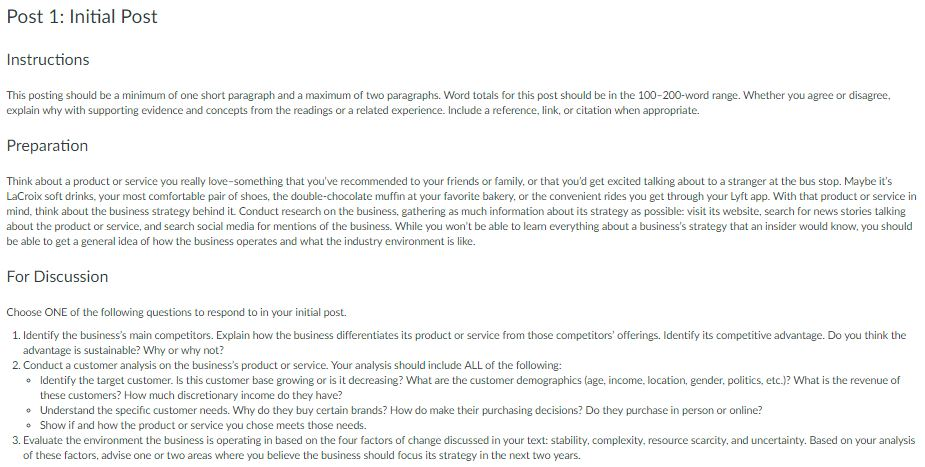This image captures a detailed instructional guide for a discussion post assignment. At the top, bolded and in a larger font, it states "Post One: Initial Post." Below this, there is a space followed by the section labeled "Instructions," which elaborates on the requirements for the post. The instructions specify that the post should be at least one short paragraph and at most two paragraphs, with a word range of 100 to 200 words. It directs participants to clearly state their agreement or disagreement along with supporting evidence and concepts from readings or personal experiences. Additionally, it notes the importance of including a reference link or citation when relevant.

The next section, titled "Preparation" in larger font, prompts users to think about a product or service they are enthusiastic about, such as LaCroix soft drinks, their most comfortable pair of shoes, a double chocolate muffin from their favorite bakery, or the convenience of Lyft rides. Users are encouraged to research the business strategy behind their chosen product or service, gathering as much information as possible.

Following another space, the "For Discussion" section appears, also in a larger font. This section instructs users to choose one of the three provided questions to respond to, based on their research and the chosen product or service. The layout is clear, with ample spacing between sections for readability.